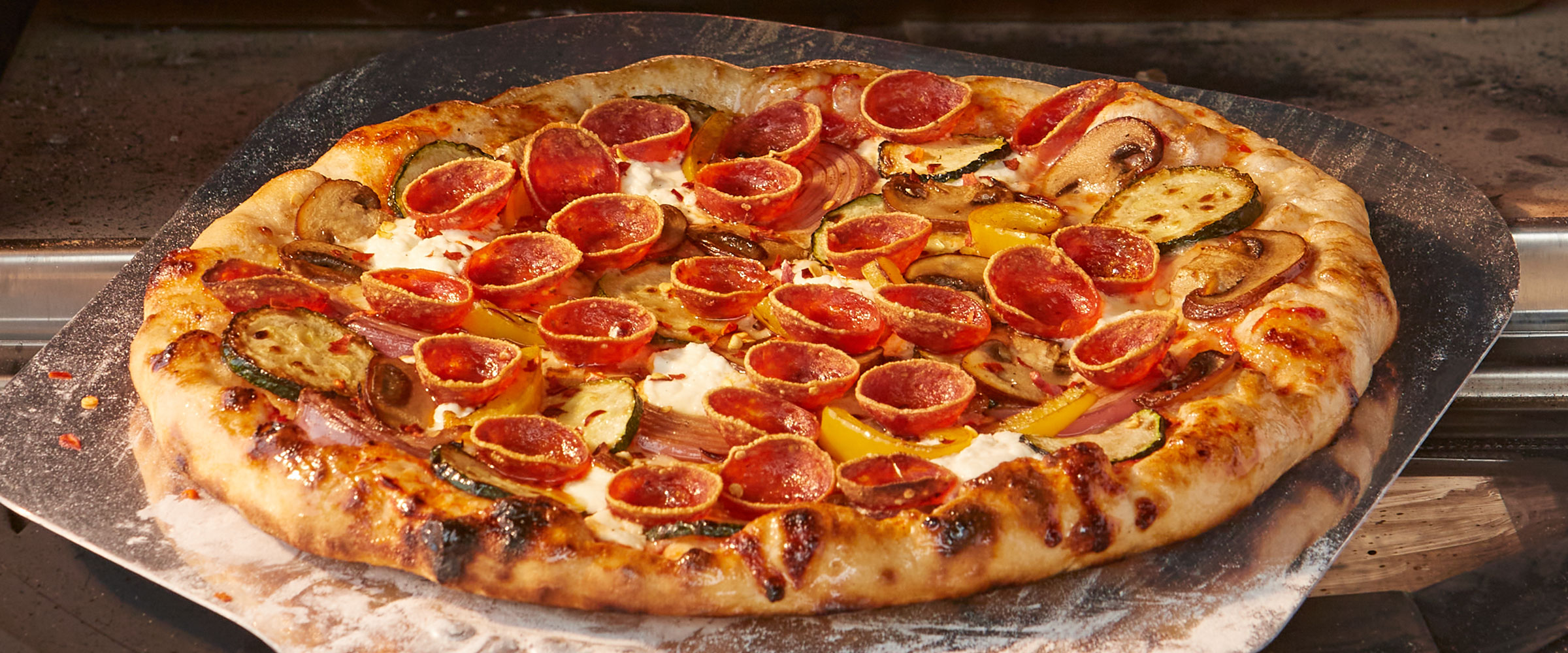This photograph captures a thick-crust pizza freshly pulled from a pizza oven, still resting on a giant metal pizza spatula. The well-cooked pizza features an array of toppings: an abundance of pepperoni that has curled into small, reddish cups, slices of green zucchini, yellow peppers, mushrooms, and onions. The crispy, browned edges of the crust and some scattered burn marks of cheese around the outer layer add to its mouth-watering appeal. The long, horizontal composition of the photo emphasizes the entire pizza, while the metal spatula beneath reflects the work of a skilled pizzaiolo.